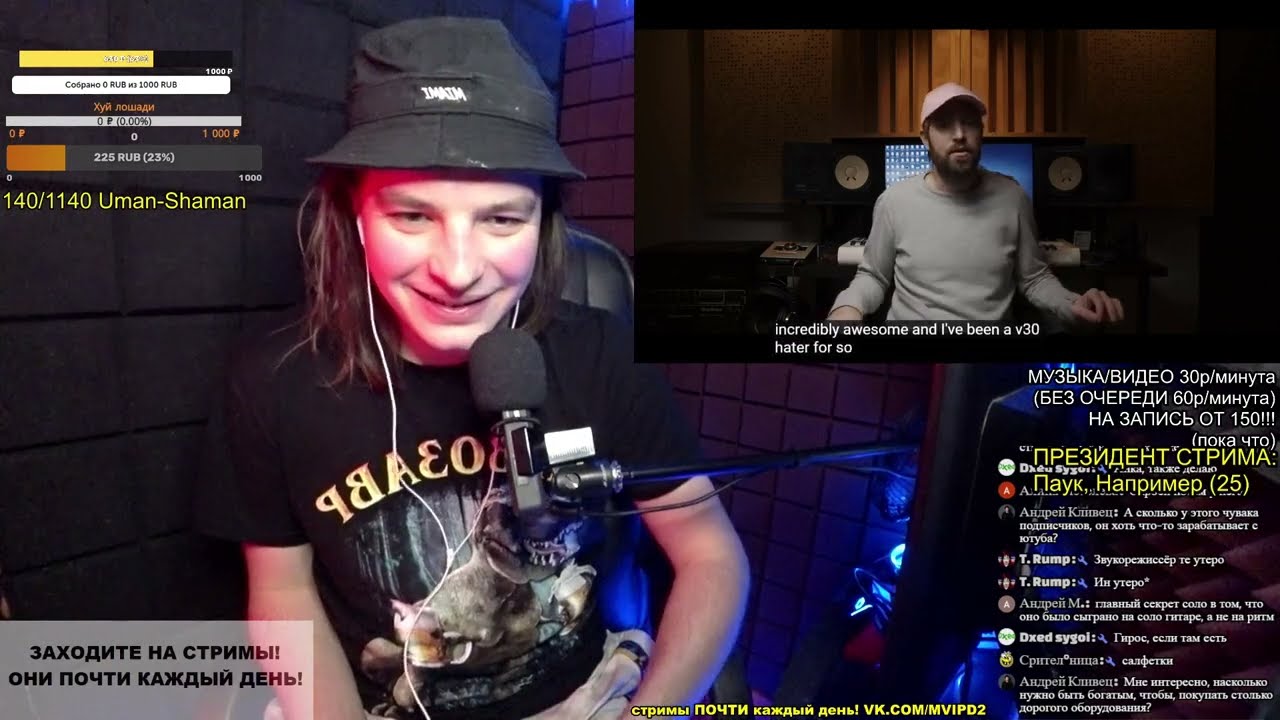This rectangular image appears to be a screenshot from a podcast or live stream session, divided into two main sections. The left, larger portion features a man with shaggy, shoulder-length brown hair wearing a stained black bucket hat. He is speaking into a microphone and sporting a short-sleeved black t-shirt with a graphic image of a rabbit and gold text above it. The background behind him resembles a stone brick wall, suggesting an indoor setting. In the upper left corner, there are donation goal bars and the numbers "140/1140" along with the text "Umen-Shaman" in yellow. The lower left corner shows some Russian text and symbols in a gray rectangular area.

On the upper right of the image, a smaller screen shows another man, seemingly in a different room with dark lighting. He is wearing a long-sleeved beige sweatshirt and a pink ball cap, with a desk and brown curtains visible behind him. He is speaking, with partially visible text at the bottom of his screen that reads, "incredibly awesome and I've been a v30 hater for so...". Both men appear to be engaging in a live broadcast or recording, adding to the dynamic nature of the scene.

In the lower right corner, there is additional text and symbols in another language (likely Russian), presented in white and yellow. The overall composition and numerous details evoke the sense of an interactive and international podcast or streaming session, with the primary color palette encompassing black, gray, beige, yellow, and various other accent colors.